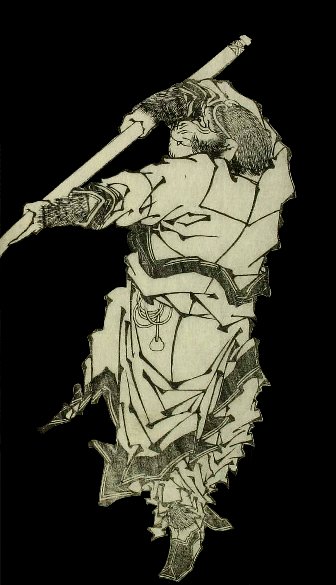This black-and-white image depicts what appears to be a simian-like figure, possibly a monkey, dressed in a stylized, layered costume or long gown with a unique pattern and frayed edges. The figure is holding a staff or javelin-like pole angled downward to the left. The creature's face is notably non-human, with a thick nose and mouth area extending from the eyes, further suggesting its animalistic nature. The intricate garment exhibits many folds and pointed details, and the figure is wearing boots, one of which is firmly on the ground while the position of the other suggests it might be up in the air. The background is entirely black, emphasizing the detailed and curious form of the figure.